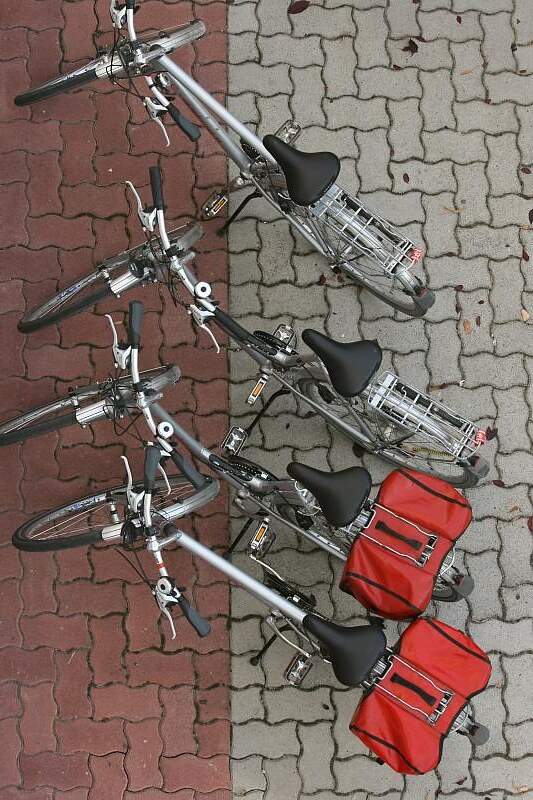This aerial photograph captures a scene of four bicycles parked on a uniquely patterned brick walkway that transitions from irregularly shaped red bricks on the left third to gray bricks on the right two-thirds. The bricks are arranged in a herringbone pattern, giving the surface a distinctive, jagged appearance. Of the four bicycles, two are black and two are silver, all featuring black seats and straight, slightly bent handlebars with brake handles. The bicycles are parked such that their back wheels rest on the gray bricks while their front wheels are on the red bricks. Each bike has orange reflectors on the pedals and red reflectors on the back. Two of the bikes, one black and one silver, are equipped with red canvas carrier bags mounted on the rear racks. The remaining bicycles have silver guards above the rear wheels, which also serve as seating areas. The arrangement of the bikes, their colors, and accessories suggest functionality, possibly for delivery, parked neatly outside what appears to be a building, as inferred by their kickstands holding them in place.